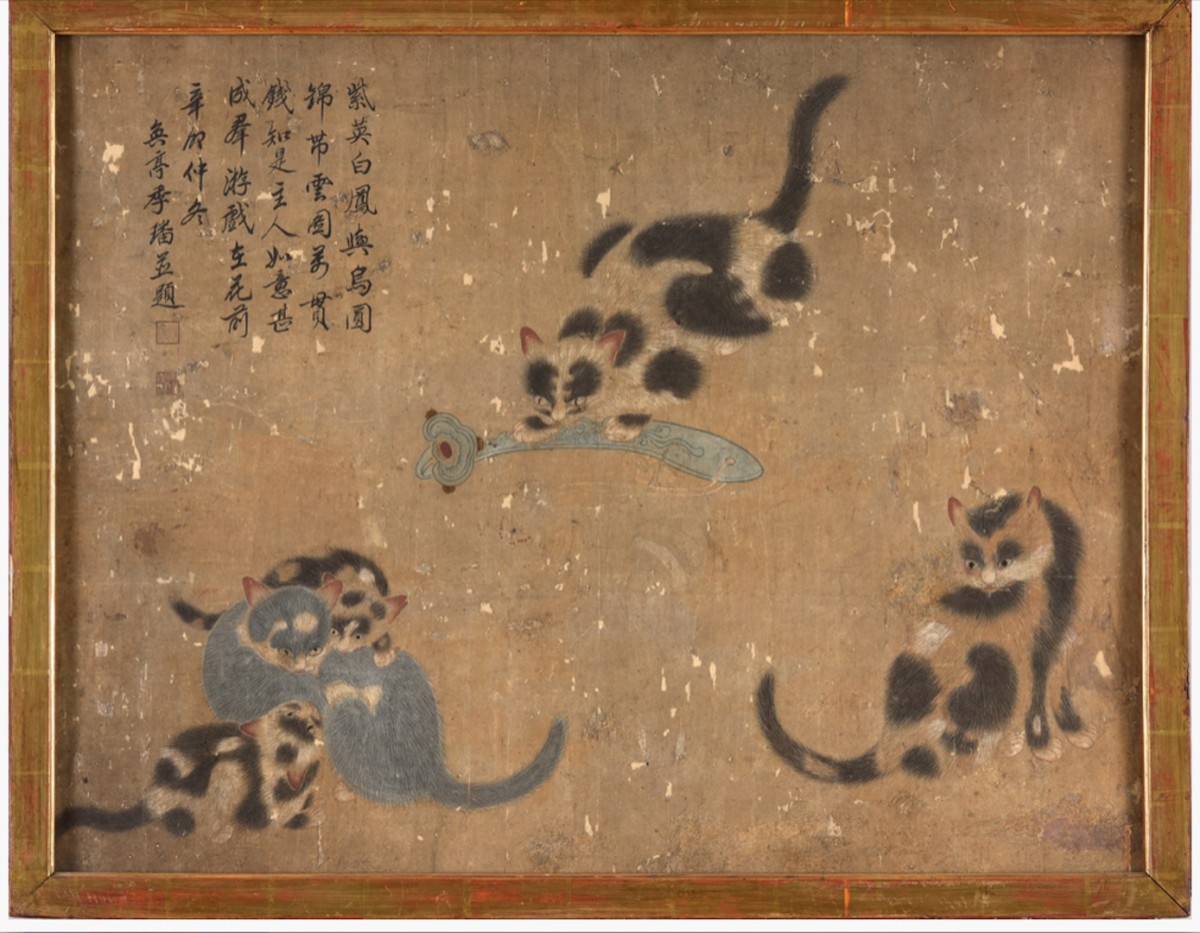The image features a detailed drawing encased in a mottled, brown timber wood frame. The brown canvas is flecked with white and adorned with an array of abstract cats in various poses, each with distinctive black and white patterns and highlighted with red accents on their ears. The top center cat, with the bushiest tail extending fur outward, is pinning down a blue object embellished with red, which resembles a fish. In the bottom right corner, a black, brown, and white cat with brown ears gazes at its reflection. The bottom left corner shows a playful trio: two small black and white cats with red-ear details and a definably outlined gray cat with additional white splotches on its head, all with raised tails. The image contains some Asian characters written vertically in black ink towards the top left, adding an exotic element to the artwork.